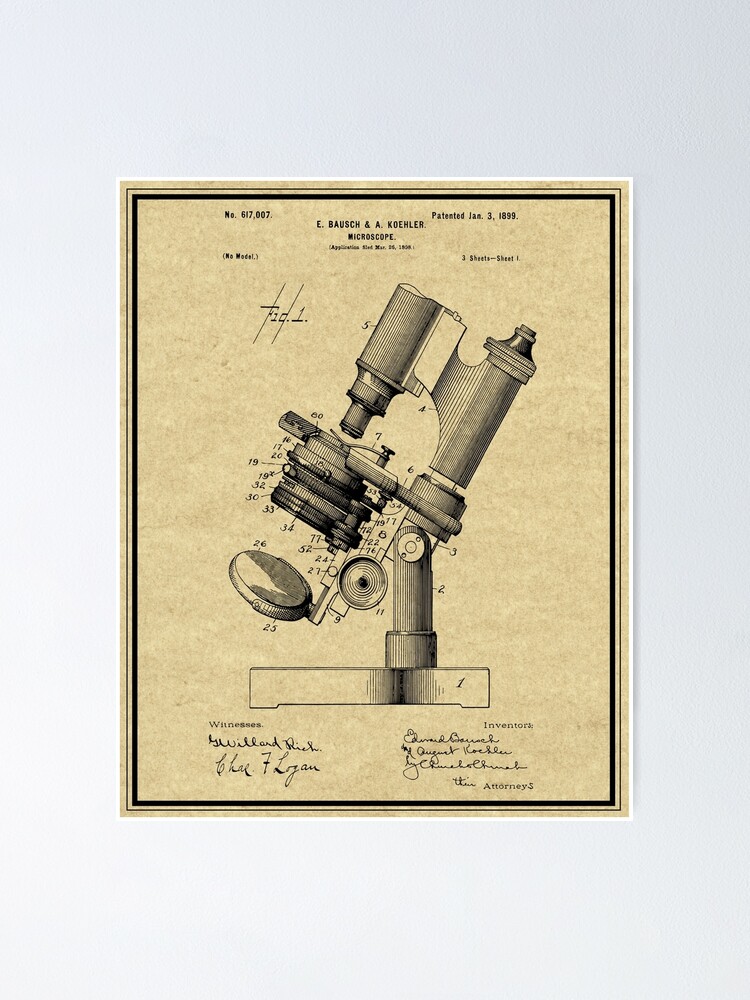The image features a detailed vintage patent sketch of a microscope design by E. Bausch and A. Kohler, prominently displayed on a discolored, peachy-brown parchment paper with a distinct black border. Centered within a white frame against a gray wall, the illustration showcases various labeled parts of the microscope, rendered in precise pen work. At the top of the parchment, the text reads "E. Bausch and A. Kohler Microscope," with the patent date "January 3, 1899" noted to the right. The left corner bears the patent number "617-007" and the words "No Model." Below the central illustration, the text "Witnesses" is on the left, accompanied by two black cursive signatures, and "Inventors" is on the right, followed by three cursive signatures. The overall appearance of the paper, including its aged and antique look, complements the historic significance of the design.